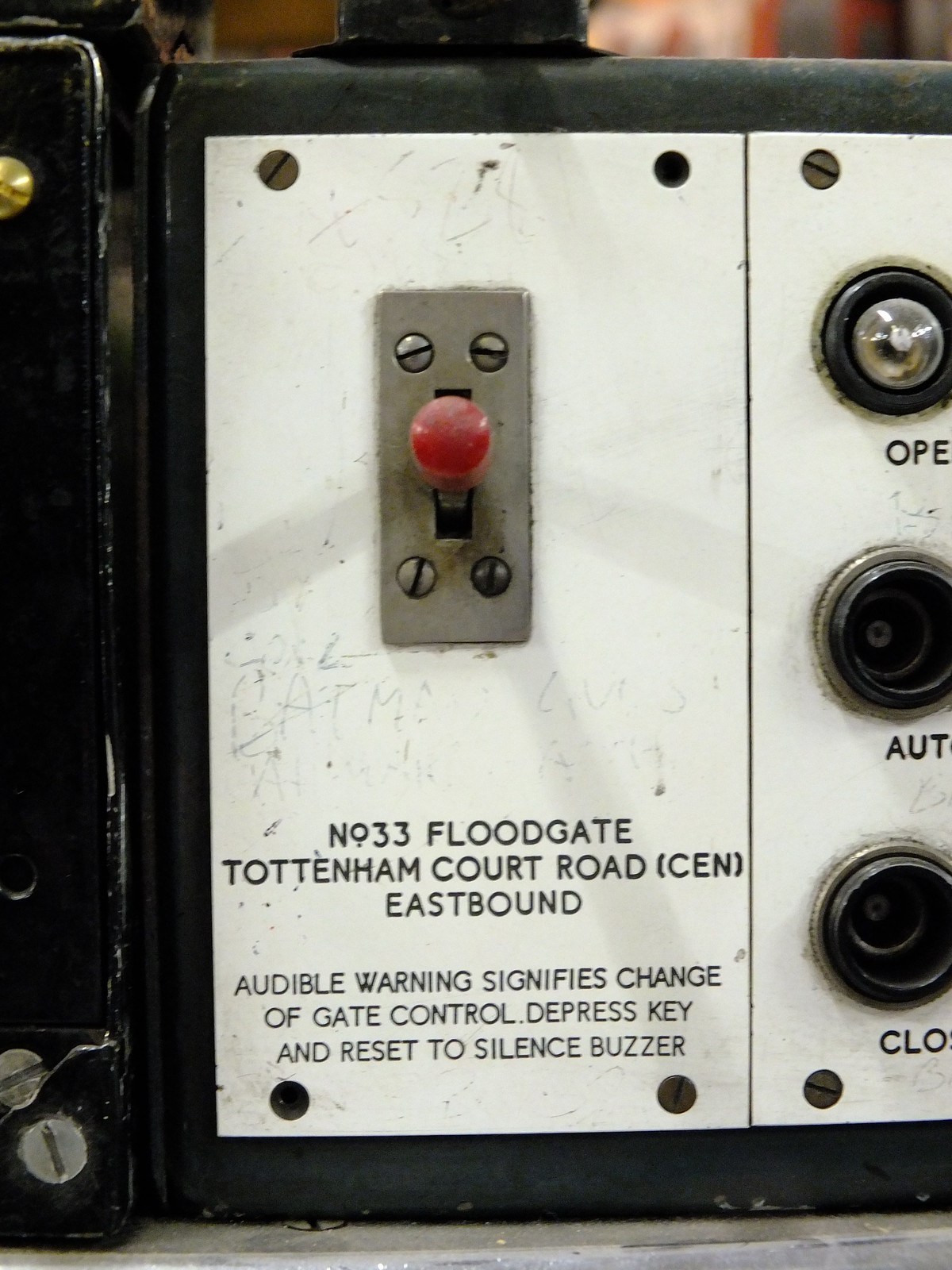The image depicts an electrical control panel partially embedded in a larger machine, which extends outside the frame to the left and right. The machine is constructed from a black material that appears to be a combination of plastic and metal, resting on a gray surface. Prominent in the image is a white rectangular plate secured to the machine by four visible screws. Centered on this plate is a silver rectangle housing a red switch. Beneath the switch, the text reads, "No. 33 Floodgate, Tottenham Court Road, CEN, eastbound." Additional text indicates, “Audible warning signifies change of gate control. Depress key and reset to silence buzzer.”

In the upper portion of the image, extending to the left corner, a partial view of a gold nub is visible. The control panel also features three small buttons to the right of the switch labeled "Open," "Auto," and "Close." The bottom left corner is adorned with the edges of silver screws, completing the intricate details of this functional machine component often found in industrial settings.